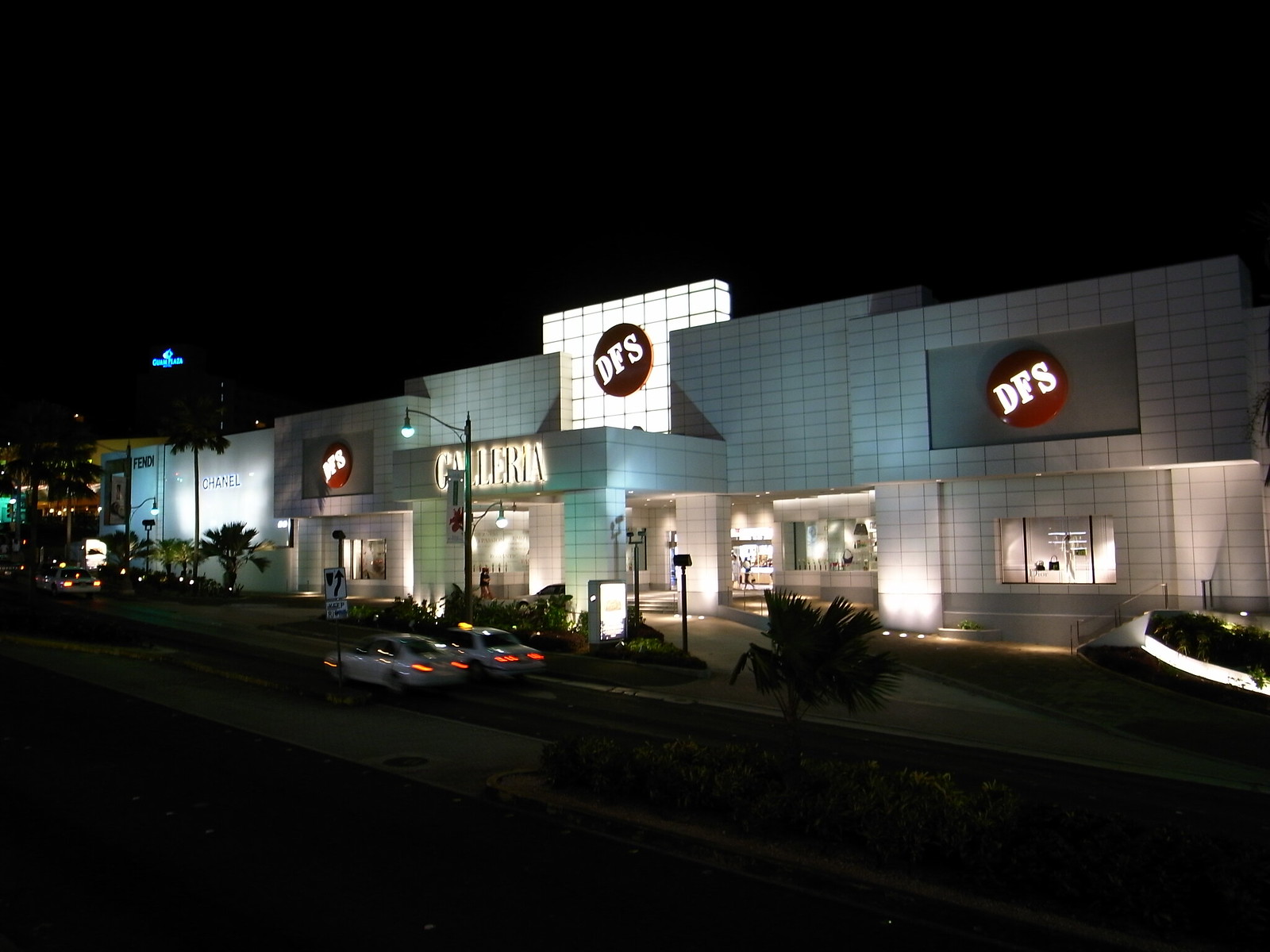This nighttime photograph captures the grand facade of an upscale shopping center known as the Galleria. The building's exterior is clad in white rectangular tiles separated by black grout, conveying a clean and modern aesthetic. Dominating the center of the image is the Galleria's main entrance, indicated by a large backlit "GALLERIA" sign in an all-caps serif font, situated on an awning that extends over a small entry porch area flanked by steps. Above this sign, centered and prominently displayed, is a circular red insignia with "DFS" in white text, a motif that repeats twice more to the sides, set against gray rectangular backgrounds.

To the left of the entrance, storefronts for upscale brands such as FENDI and CHANEL are visible, signaling high-end retail offerings. The multi-story building features windows only on its lower level, further highlighting the retail space. The scene also reveals practical details: a stoplight stands in front of the Galleria, and three white cars with their lights on are halted nearby, brake lights gleaming against the dark night. The foreground includes some landscaping with short palm-style trees and illuminated patches of foliage, contributing to the exclusive ambiance. Emphasizing the vibrant environment, two people are seen walking into the entrance, underlining the active nightlife at this sophisticated mall.